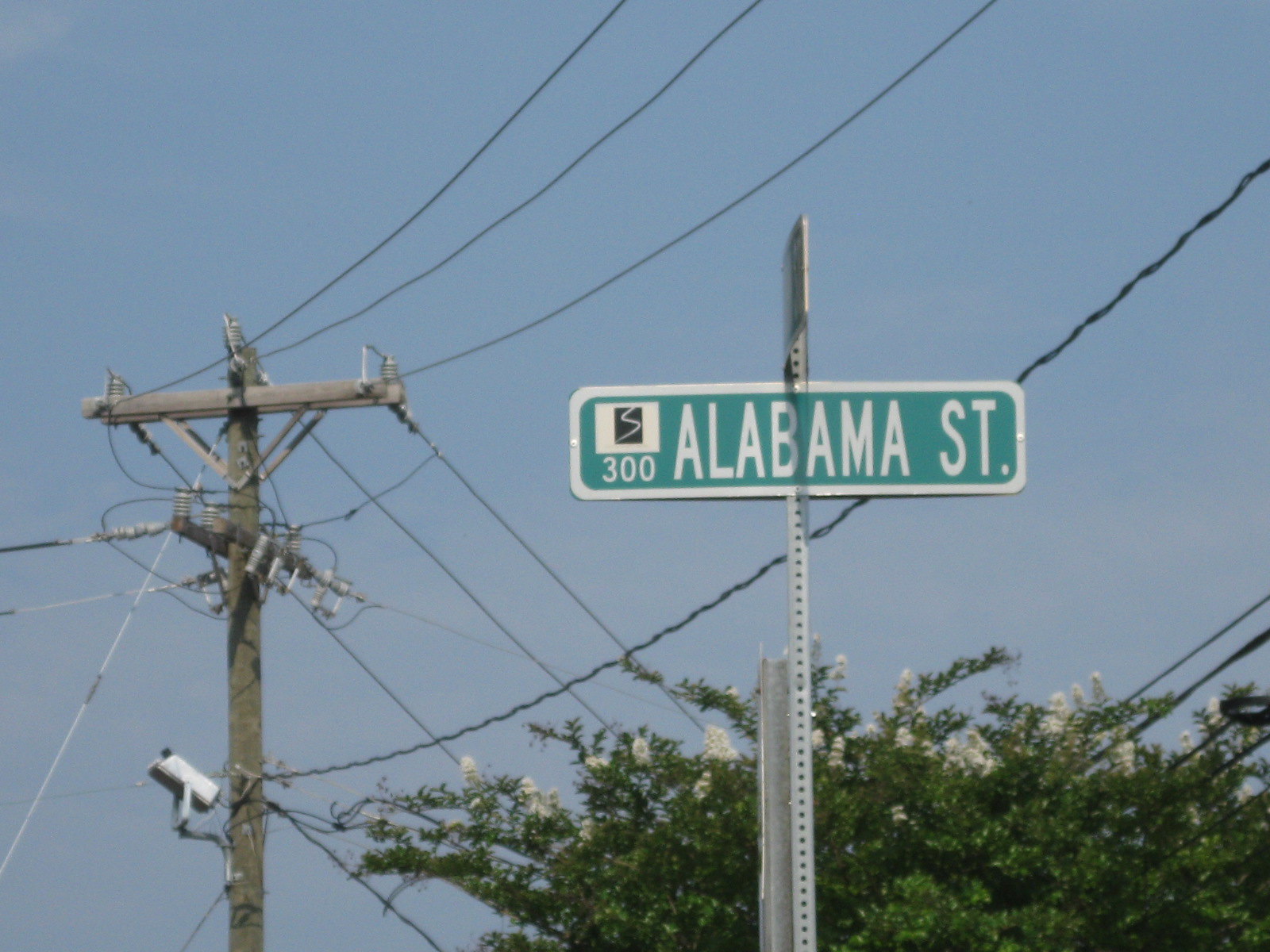This color photograph captures an upward view of a road sign against a blue-grey sky. Positioned in the center of the image, the road sign is mounted on a grey pole and is outlined with a white border. The main background of the sign is green, featuring a white rectangular section in the upper left corner with a small black square containing a white "S" symbol. The primary text on the sign is white and reads "300 Alabama Street."

To the left of the frame stands an electricity pole, from which numerous power lines fan out, criss-crossing the sky above. Beneath the sign, toward the center and right, the tops of lush bushes are visible, with what appear to be small white flowers adorning their edges. Though the sky might have some wisps of cloud, it is somewhat ambiguous due to what could be photographic artifacts not present on the lower branches.